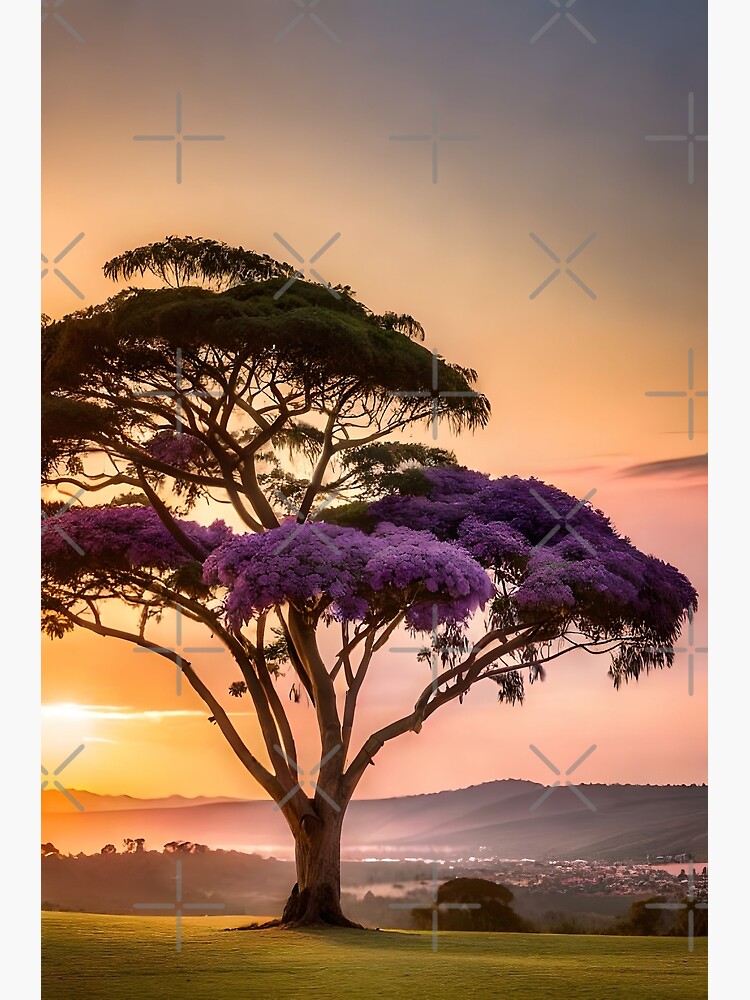In the image, a magnificent tree stands prominently in the center of a neatly mowed grass field. The tree's thick trunk supports an expansive canopy that unfolds in two distinct layers. The lower branches are adorned with clusters of light purple flowers, creating a vibrant contrast against the deep green leaves of the upper canopy, which appear darker due to the shade. The setting sun to the left casts a warm glow of orange and purple hues across the sky, illuminating the tall, distant mountainous hills. Below the hills, nestled in a valley, a small city with minuscule buildings is visible, enhancing the picturesque scene. Additionally, a tranquil lake can be seen in the landscape, contributing to the serene ambiance of the scene.